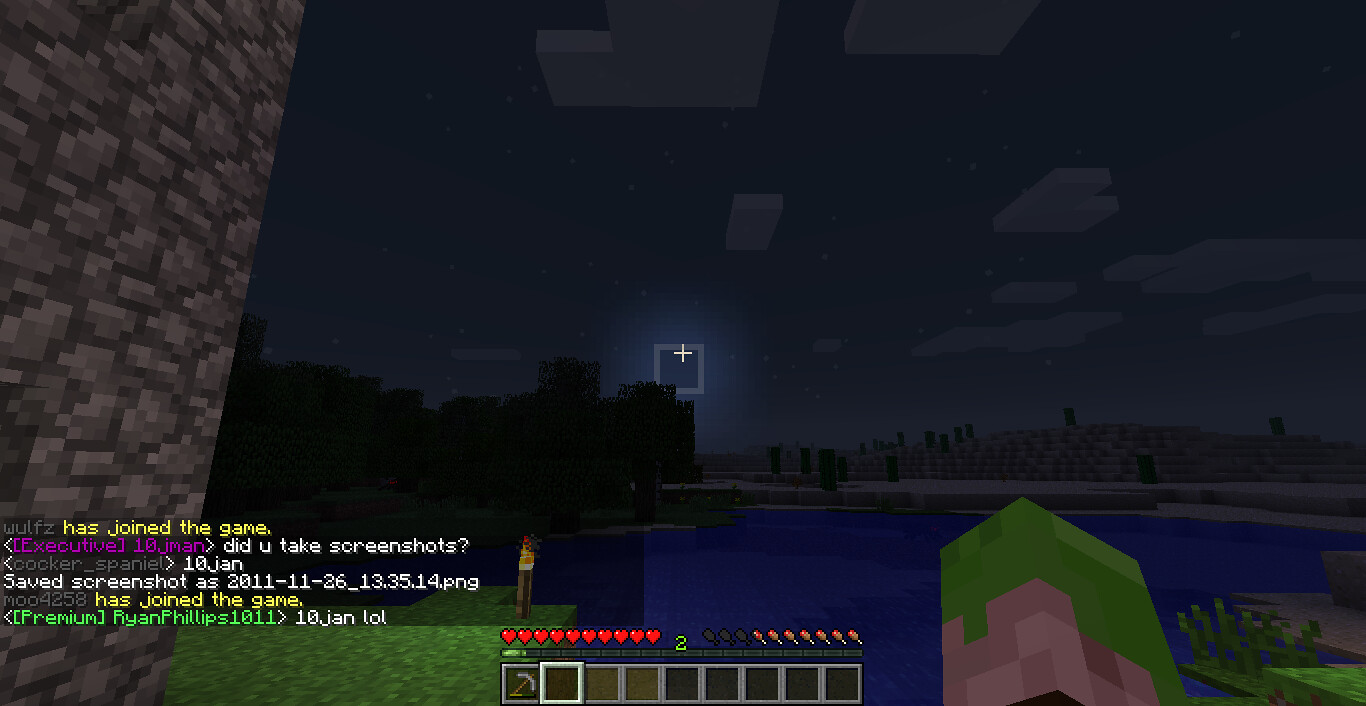This detailed Minecraft screenshot captures a nighttime scene where the player stands on a grassy terrain by a body of water. To the left, there's a desert landscape marked by cacti and sand, while to the right, a staircase ascends. In the foreground, the player is highlighted with a white cursor at the center of the image, aiming towards the glowing moon in the deep indigo sky, which features pixelated grayish-blue clouds. A wall of cobblestone rendered in mauve, beige, brown, and black is visible on the left. The player's health is fully intact, with red hearts displayed, and they are at XP level 2, missing three hunger bars, symbolized by translucent 'lollipop' icons. They wield a stone pickaxe, already at half durability. The multiplayer aspect of the game is evident by the multicolored chat texts displayed at the bottom left, with messages indicating the logins and interactions of various players such as Wolfs, executive 10jman, Walker_Spaniel, Moo4258, and PremiumRyanPhillips1011, capturing a lively moment within the server. The screenshot is timestamped November 26, 2011, at 13:35, saved as a PNG file.